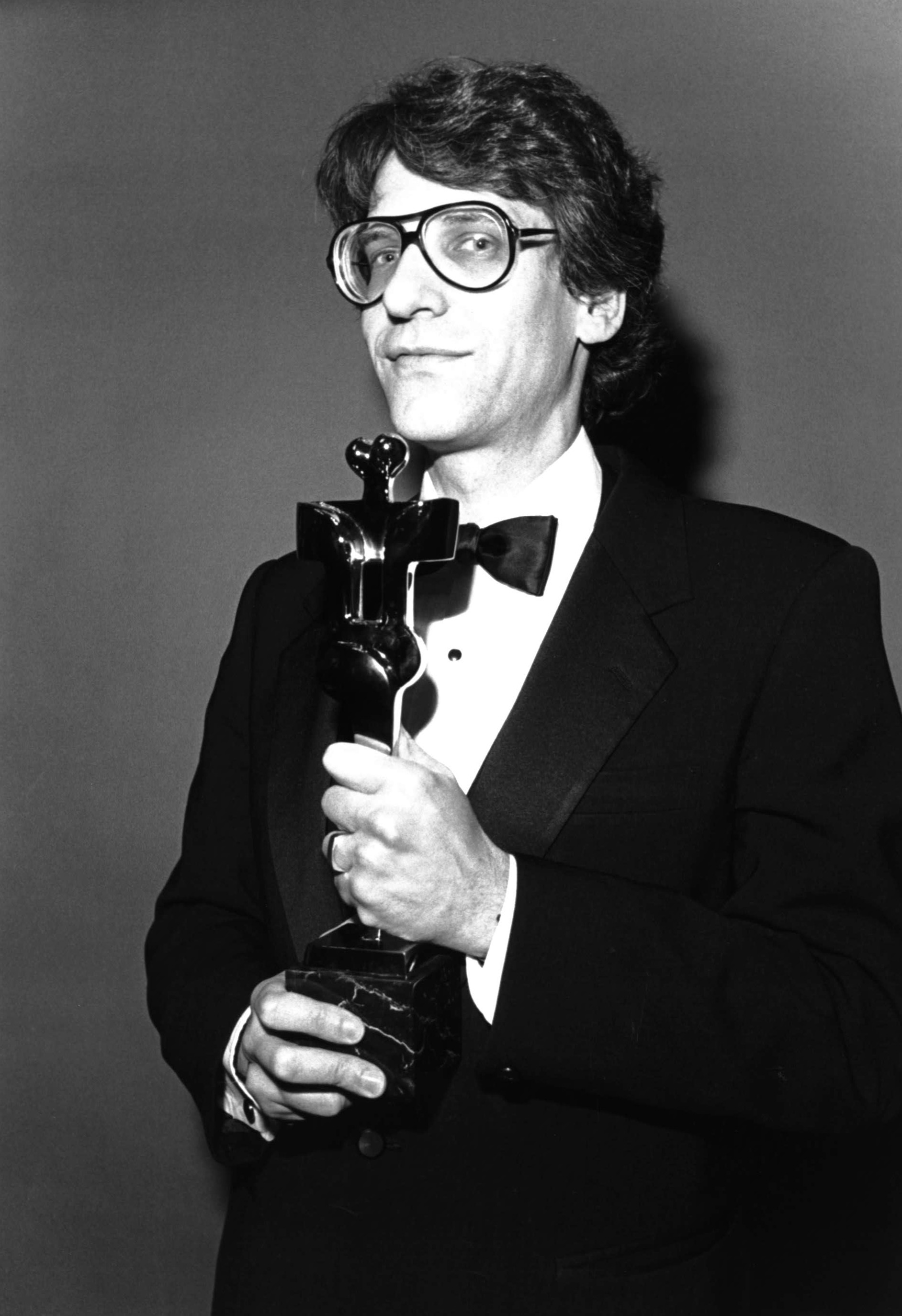This black-and-white photograph from the 1980s captures a waist-up portrait of a man wearing a black tuxedo with a white collared shirt and a black bow tie. His hair is short, wavy, and neatly parted to the side, feathering slightly over his ears and curving down to the back of his neck. He has black-rimmed glasses with a bar across the top and another over the bridge of his nose. The man is holding an abstract award or statue, composed of a black stone base and a possibly gold top, with his right hand on the base and his left hand on the middle section. A ring can be seen on one of his fingers. The background is a plain, grayish wall, likely a different color in reality. The overall setting suggests an award ceremony.